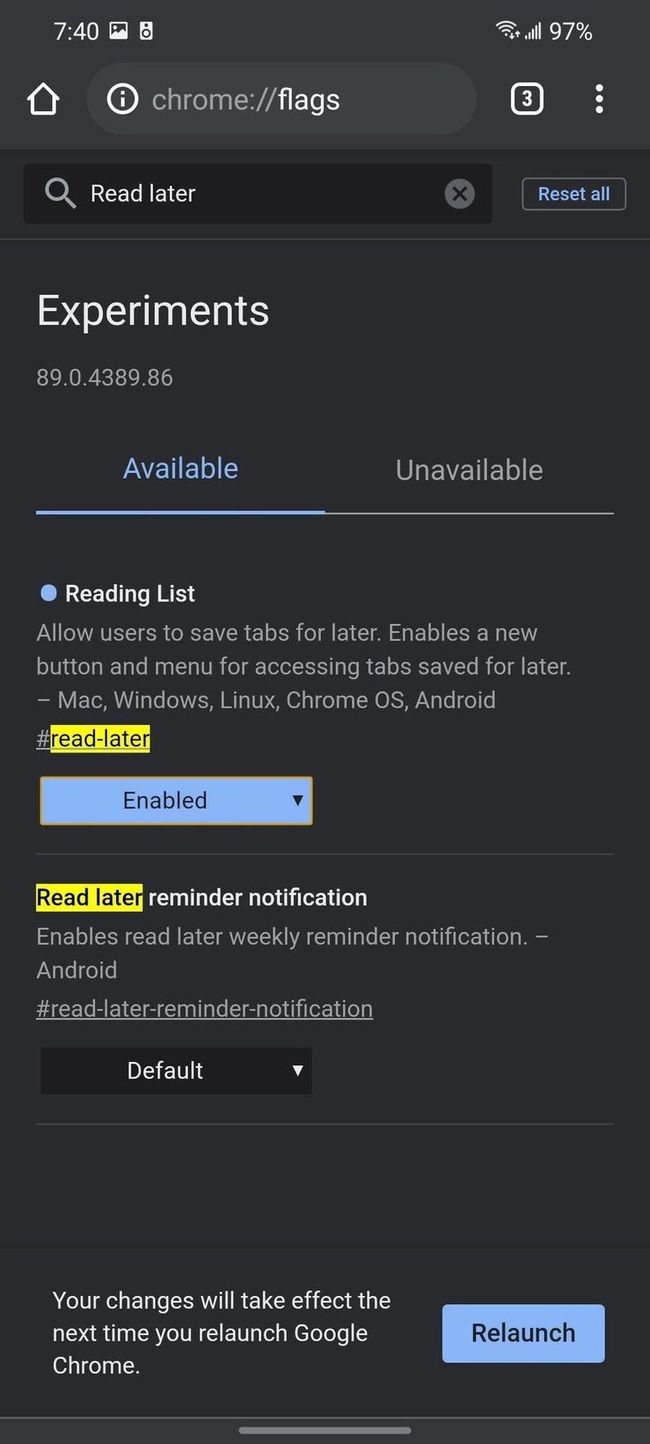The image displays the mobile version of Google Chrome's flags settings page. At the top of the screen, there is a navigation bar featuring a home button on the left, an address bar in the center displaying "chrome://flags", and a tabs button on the right indicating three open tabs. Below the navigation bar, there is a search bar with the text "read later" typed into it, and a "Reset all" button to the right.

The main content area is titled "Experiments" with the version number "89.0.4389.86" beneath it. This section is divided into two tabs: "Available" and "Unavailable." The "Available" tab is selected, and it highlights two specific features:

1. **Reading List**: This feature allows users to save tabs for later access. It mentions that it enables a new button and menu for managing these saved tabs across multiple platforms including Mac, Windows, Linux, Chrome OS, and Android. The feature is tagged with "#read-later" and is enabled.

2. **Read Later Reminder Notification**: This feature enables weekly reminder notifications for the read later list and is specific to Android. It is tagged with "#read-later-reminder-notification" and set to the default setting in a dropdown box.

There is also a "Relaunch" button at the bottom of the page, which restarts the app to apply any changes made to these settings.